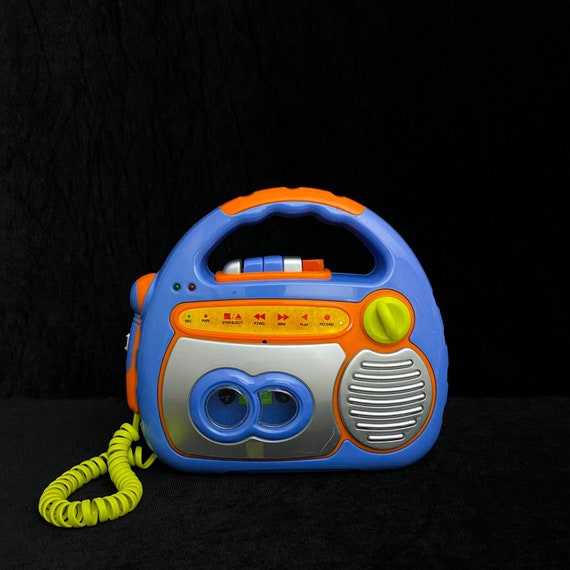This image showcases a child's cassette player radio set against a stark black background, slightly revealing the toy's edges due to a very slightly lighter black surface. The toy's main body is blue, accented with orange highlights, and it features a convenient handle on top. The design includes a distinctive microphone mounted on the side, which is primarily red and blue, connected by a coiled yellow telephone-style cord, indicating that the toy can also function as a PA system.

On the toy's front, a silver grill covers the speaker section, accompanied by a silver and blue cassette compartment with visible blue circles. The array of buttons on top includes specific colors: two blue, two white, one red, and one orange, designed for various functions such as stop, eject, fast forward, play, rewind, and record. A green volume knob is situated on the front right for easy control. This detailed toy demonstrates a fun and interactive way for children to engage with audio playback and recording.